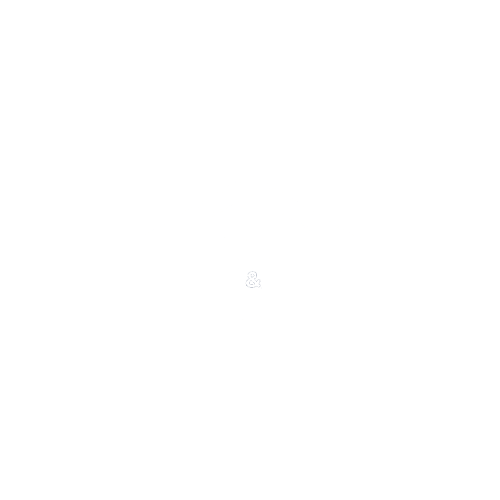A completely blank white screen is depicted in this image, possibly indicating an error or glitch. The top of the screen features a "flag" button, suggesting that the user can report or mark the error. This white screen represents common occurrences on the internet when pages fail to load. Such instances can result from a variety of issues, including server downtime, connectivity problems, or even external factors like adverse weather conditions or power outages. Additionally, website overloads due to high traffic or deliberate downtime can also cause this blank display. Overall, this image encapsulates the occasional unpredictability and technical challenges of browsing the internet.